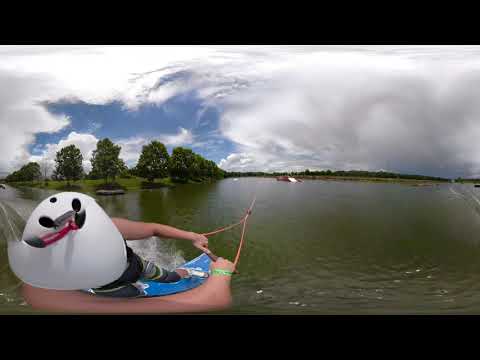The panoramic image, taken from the helmet of a person wake surfing, provides a dynamic view from the water. The surfer is wearing a white helmet, a sleeveless dark shirt, and dark sweatpants, with a distinctive green strip on their right arm. The camera's position, mounted on their head, captures arms extended to hold a light reddish rope, presumably connected to a distant boat that is not visible in the shot. The surfer's blue wakeboard is prominently visible as they navigate a red ramp positioned in the center of the frame.

The lower left part of the image shows part of the surfer's lower body and arms, enhancing the immersive feeling of the shot. Surrounding the surfer, the water appears greenish, bordered by a grassy bank with trees lining the shore on the left. Additional greenery and bushy areas can be seen on the far right and further into the distance. 

The sky, which takes up the top portion of the image, is predominantly covered with clouds, leaving only about 20% of it blue and clear. The overall distorted nature of the image adds to the sense of movement and action, documenting the thrilling experience of wake surfing.